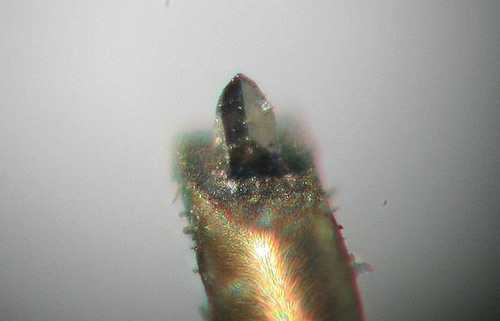The image features a predominantly silver metallic object, which appears hollow and cylindrical, set against a gradient grayish-purple background that fades from darker shades at the bottom to lighter whites and purples at the top. Emerging from the top of this cylindrical structure is a black object, likely rectangular and slightly tilted, which seems to be either resting on or extruding from the silver form. The metallic surface is adorned with various bubbles or beads, suggesting it could be underwater, as these elements appear to be gathering around it. The metallic object has a brass tone with hints of green and blue, possibly indicating the presence of copper, and exhibits a textured, somewhat hairy appearance. Additionally, a triangular chunk of metal juts out from the base of the structure, enhancing its abstract and intriguing aesthetic.